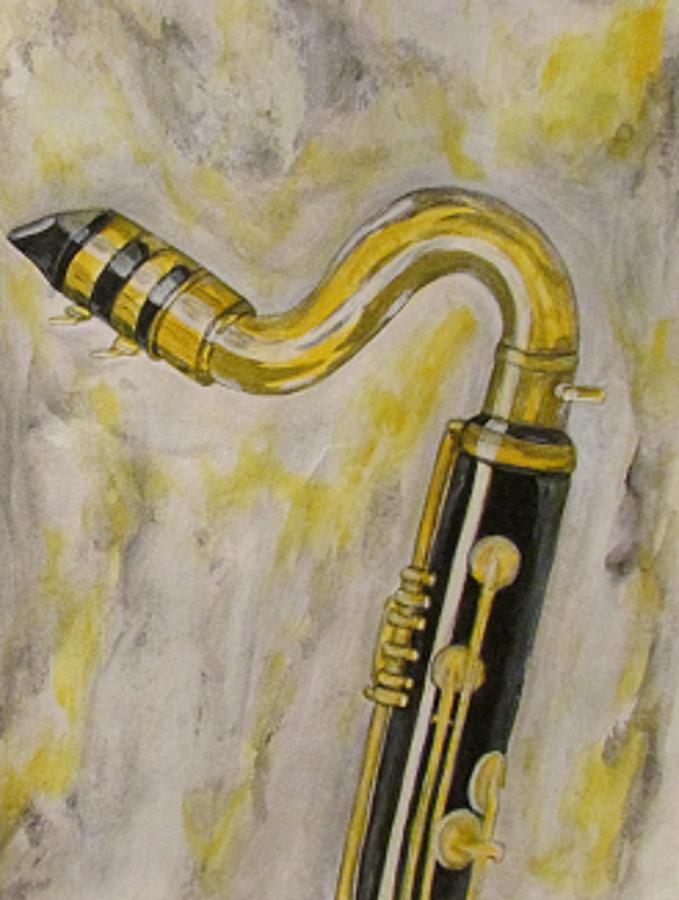This painting, set within a vertically aligned rectangular frame, showcases an instrument that appears to be a clarinet or possibly a saxophone, primarily characterized by its intricate details and striking colors. The focal point is the mouthpiece, located in the upper left corner, which features alternating bands of black and gold. This mouthpiece is attached to a curved golden stem that transitions into a larger black cylindrical body adorned with gold buttons and keys. 

The instrument's body arcs gracefully before extending straight down the image, but its bottom section is not visible as it extends beyond the image's lower edge. The background of this watercolor artwork consists of textured smears and strokes in shades of light brown, gold, dark brown, gray, and subtle hints of yellow and purple. These blended tones give the composition a dynamic yet harmonious feel, with the light brown being the dominant color. Every brushstroke seems to merge seamlessly, creating a visually compelling backdrop that complements the elegant depiction of the instrument.